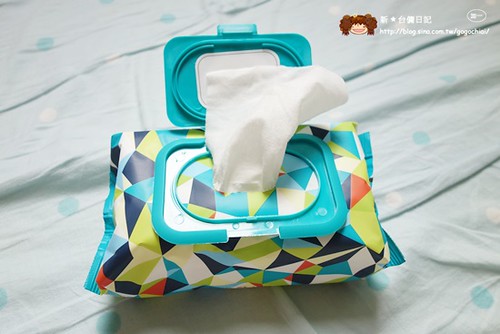This image features a meticulously arranged scene showcasing a pack of baby wipes centrally positioned, captured on a flat surface that could either be a table adorned with a tablecloth or a bed with a bed sheet. The setting appears to be indoors, potentially inside a baby's room. The focal point is an open pack of baby wipes, with one wipe partially pulled out from a slot on top. The packaging of the wipes is made of plastic and displays a vibrant design of various triangular and trapezoidal shapes in colors including dark blue, light blue, light green, white, and an orange-red hue. 

In the top right corner of the image, there is a discernible logo depicting a girl with brown hair accompanied by some Asian lettering, possibly Chinese, and a small, unreadable website address. Notably, there is no recognizable brand name or readable text on the packaging. The light spectrum in the image showcases colors of gray, light blue, white, orange, black, light green, white, and brown, adding to the scene's detailed composition.